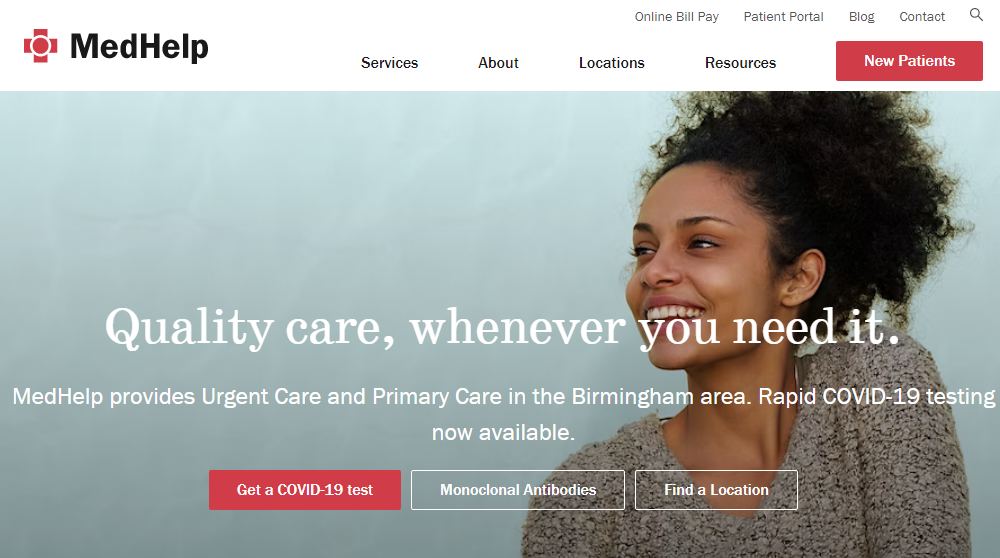This screenshot captures a medical website in landscape mode. In the upper right-hand corner, there are navigational options including "Online Bill Pay," "Patient Portal," "Blog," and a search bar. This layout indicates that the site provides various patient-oriented services. The upper left-hand corner features the logo, which consists of a red square cross with a circle in the middle and the bold text "Med Help" in black.

Below the logo are tabs for "Services," "About," "Locations," and "Resources," as well as a prominent red button labeled "New Patients." The center of the screenshot is dominated by a large photograph set against a very light teal background. On the right side of this visual, a dark-skinned female model with vibrant, fluffy hair and a stylish sweater smiles warmly.

Overlaid in white font are the words "Quality care whenever you need it." Below this, additional text reads "Med Help provides urgent care and primary care in the Birmingham area. Rapid COVID-19 testing now available." Beneath this message are three buttons: a red one labeled "Get a COVID-19 test," and two clear buttons labeled "Monoclonal Antibodies" and "Find a Location," respectively.